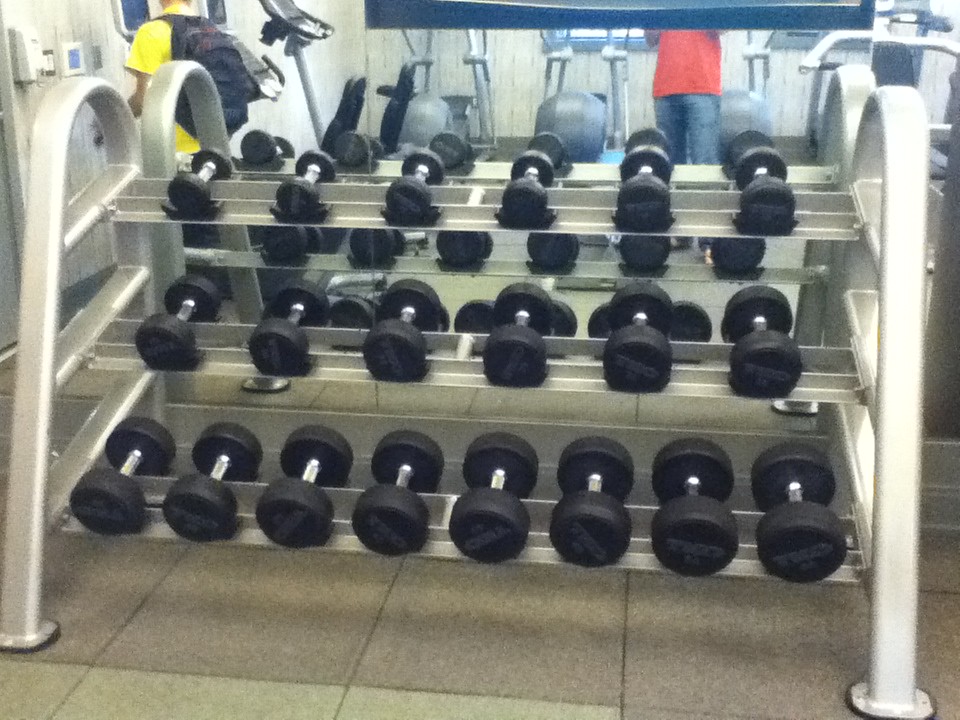This image depicts a gym setting with a prominent three-tiered rack of dumbbell weights in the foreground. The weights are organized by size, with the heaviest positioned on the bottom tier and progressively lighter weights on the middle and top tiers. The rack itself features arched silver supports on the ends and clear plastic shelves to hold the weights. The heaviest weights appear to be around 25 pounds, with intermediate weights of 10-15 pounds in the middle, and the lightest weights—some as little as 5 pounds—on the top.

In the background, various exercise machines such as treadmills, ellipticals, and possibly stationary bikes are visible, indicating a typical workout area. The room has an off-white, tiled floor, and the left wall is equipped with apparatuses, including a sanitary dispenser and a thermostat.

Also visible are two individuals; one on the left wearing a yellow shirt and a black backpack, and another on the right dressed in a red shirt and blue jeans. These individuals are casually positioned within the gym, adding a sense of activity to the scene.